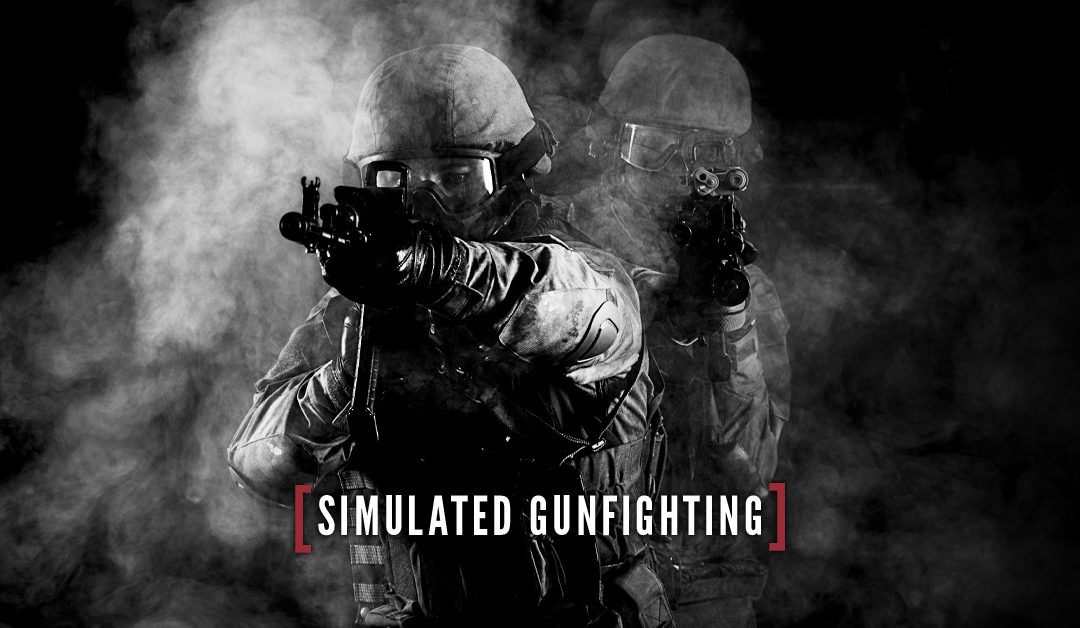This black and white photograph captures an intense moment between two soldiers geared in full military combat attire. From helmets and goggles to thick jackets, vests, and black gloves, they are equipped from head to toe in tactical gear. Each soldier holds a rifle pointed directly at the viewer, with one soldier positioned behind and slightly to the right of the other. The photograph has a dramatic horizontal composition, roughly twice as wide as it is tall, and features dense white smoke predominantly on the left side, partially obscuring the men. The scene is framed by a dark background, enhancing the stark contrast of their gear and the smoke. At the bottom of the image, white block text reads "SIMULATED GUNFIGHTING" enclosed within red brackets, adding to the graphic, intense feel of the photograph.